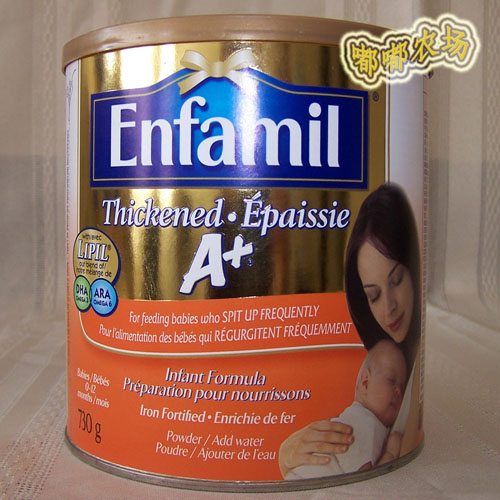This is a close-up photograph of an Enfamil infant formula can, designed specifically for babies who spit up frequently. The can is cylindrical with a white main body, featuring a removable brown plastic top. The front half of the can is split into two distinct color sections: the upper portion is gold with "Enfamil" written in white lettering, while the lower portion is orange with additional information.

At the top right corner of the can, there is a series of four Asian characters, likely Japanese or Chinese. The label prominently features the text "Thickened" and "épaissie" (French for "thickened"), followed by "A+." An orange banner at the bottom reads, "for feeding babies who spit up frequently," repeated in both English and French, along with "infant formula" and "préparation pour nourrissons." It states the content as "Iron fortified, powder, add water" and specifies the weight as 730 grams.

A detailed illustration on the bottom right of the can depicts a mother of European descent with long brown hair, lovingly holding her sleeping baby, who is wearing a white t-shirt, against her chest. The mother's eyes are cast downwards as she comforts her child. The background of the photo is a white surface with a subtle patterned texture, somewhat resembling fabric or the inside of a microwave.